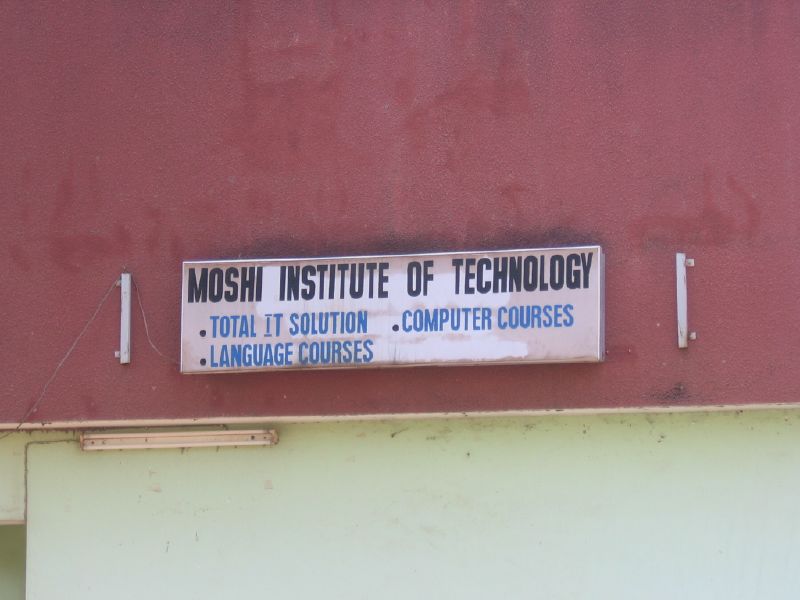The photograph depicts a close-up view of a dilapidated sign on the side of a building, taken outdoors during the daytime. The background features a medium brownish-red, slightly pixelated wall, possibly painted cement, which makes up the top two-thirds of the image. This red section overhangs a dull, light green lower section that appears rather dirty, with visible cobwebs and possibly bugs. Hanging just below the red overhang is a fluorescent light, and there may also be other lights or power sources around the sign. The sign itself is a weathered, faded white with black lettering that reads "Moshi Institute of Technology." Beneath this, in medium blue text, are the bullet points: "Total IT Solution," "Computer Courses," and "Language Courses." The sign appears to have been designed to light up at one time, and there are brackets or tie-downs on either side, potentially for supporting larger signs. Below the sign, we can slightly see the top of a worn-down, rusted white door with chipped paint.